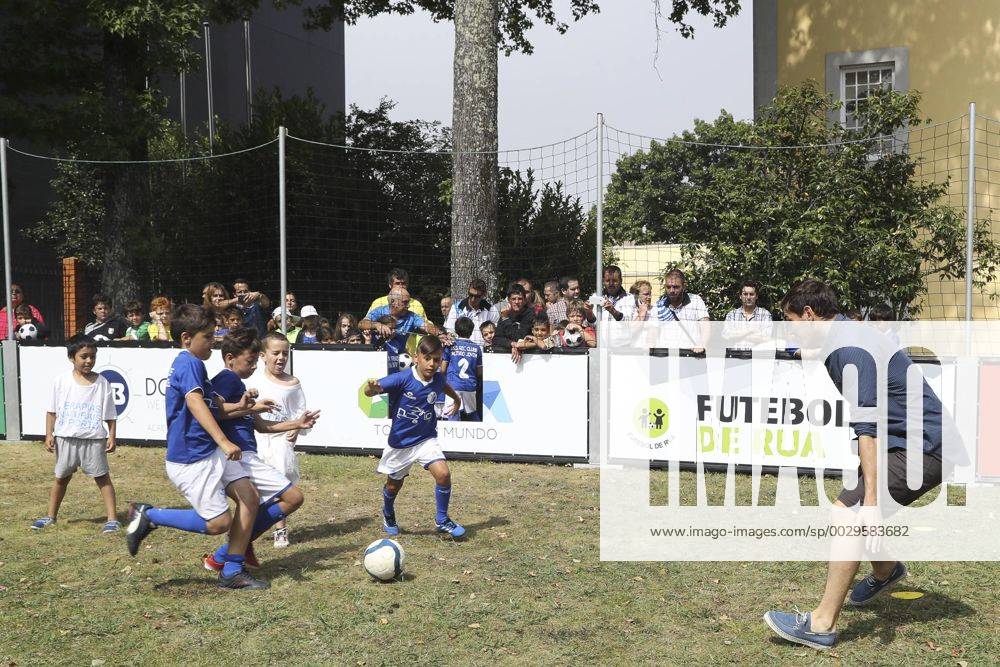The image depicts a group of young children, approximately four to six years old, playing soccer on a grassy field. Positioned near the bottom of the image, the children are actively kicking a soccer ball towards a partially obscured goaltender, who appears larger than the other players. The children are dressed in blue jerseys, white shorts, and long blue socks, with matching blue soccer shoes. Surrounding the field is a white fence, designed to prevent the ball from leaving the area, and beyond it, there are numerous spectators, likely comprising families, friends, and other children watching attentively. A watermark labeled "image" is prominently displayed above the goaltender, partially obstructing the view. The background reveals a mix of natural elements, including trees and bushes, as well as several large, dark-colored structures that could be schools or other buildings. The atmosphere suggests a community gathering, with spectators close to the field and a taller fence safeguarding them from stray balls.